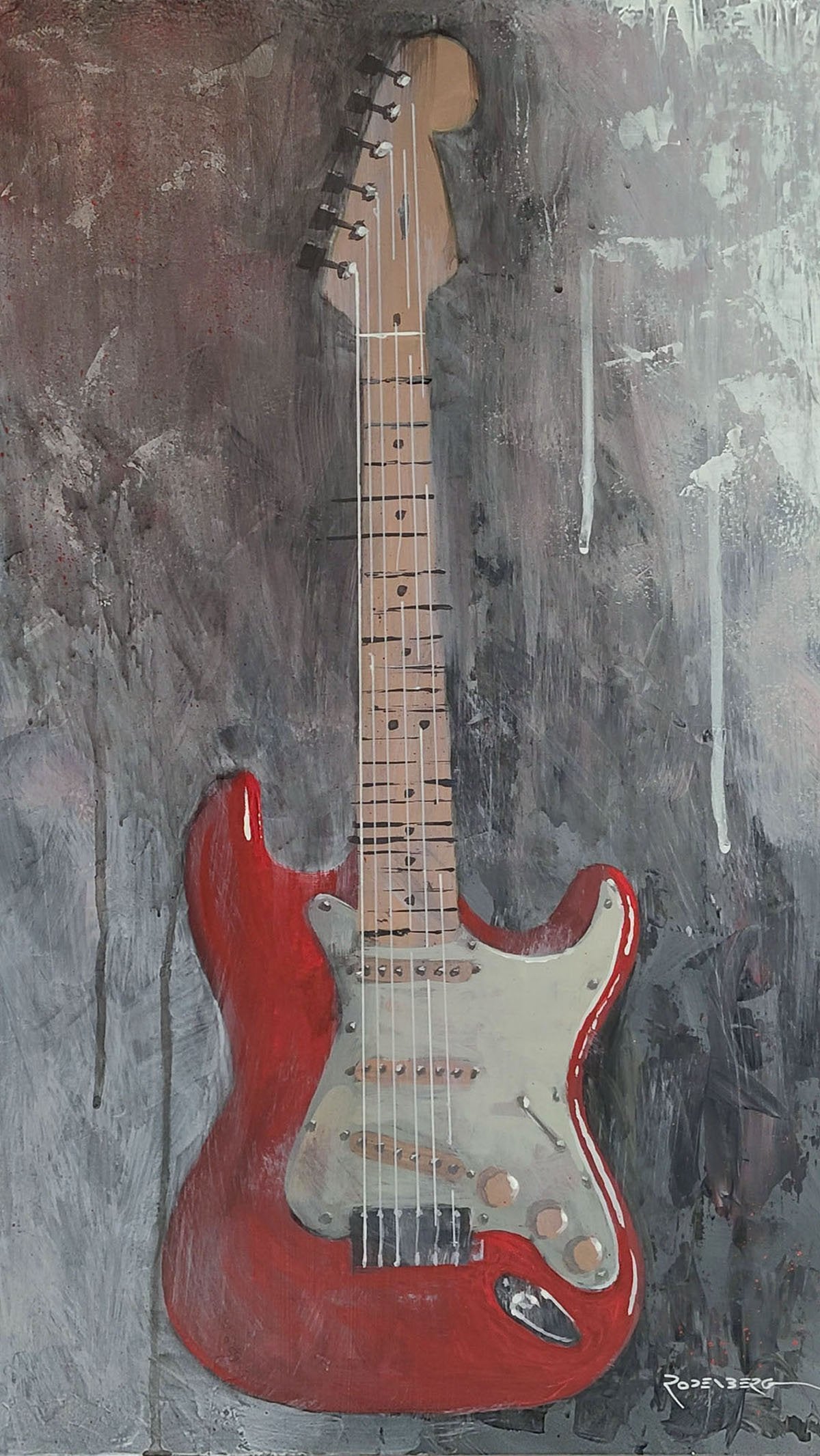This is a detailed painting of a red guitar, prominently featured against a dark, graffiti-style background with white and black elements. The guitar has a standout white faceplate and distinct gold elements, including the arm where the strings are attached. The six strings appear to have a pinkish hue that seems to complement the reddish wooden tones of the guitar. The background, although predominantly black, has patches of white shining through, adding to the overall contrast and depth. The bottom right corner of the painting features a signature or name, likely Rodenburg, despite being somewhat illegible. The entire composition focuses solely on the vertical arrangement of the guitar, making it the central and only subject of the artwork.